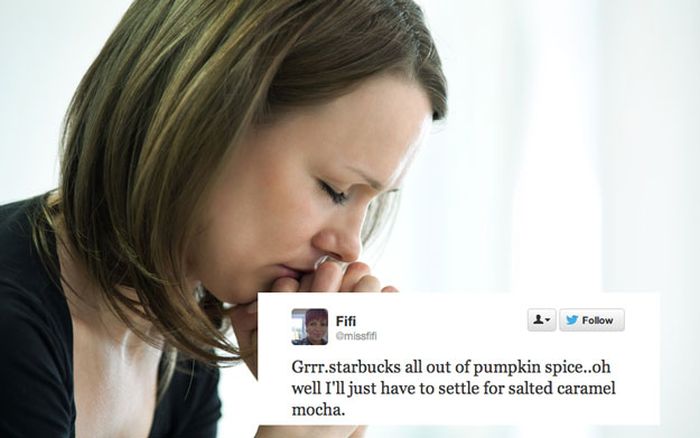The image prominently features a despondent-looking woman positioned on the left side, with a close-up profile showing her short blonde hair styled in a bob. She is wearing a black shirt and has her eyes closed, head bowed, and hands clasped together in a prayer-like position under her nose, conveying a deep sense of sadness or disappointment. The background is primarily white, with a faint white stripe visible on the right-hand side, and a set of light-filtering white curtains in the background, adding to the overall somber tone. In the bottom right corner of the image, there is a screenshot of a tweet from a user named Fifi (@MissyFifi), accompanied by Fifi's logo and handle, and options to view the profile or follow. The tweet reads, "Grrr, Starbucks all out of pumpkin spice. Oh well, I'll just have to settle for salted caramel mocha." The woman in the image does not resemble Fifi, suggesting that the image and tweet are juxtaposed for humorous or meme-like effect.